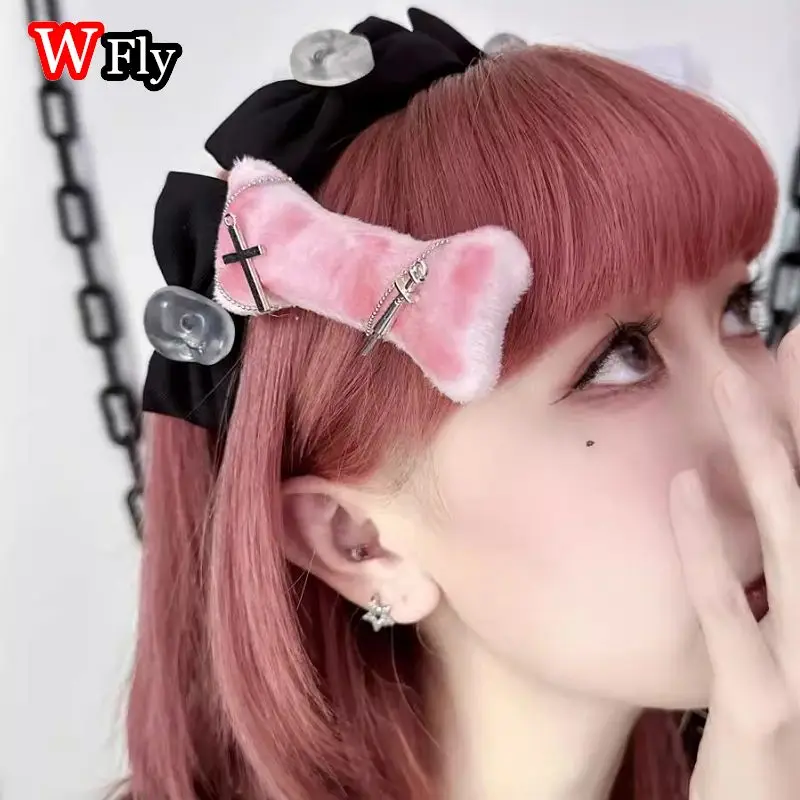This is a close-up photograph of a young Asian woman with red hair, partially obscured by her raised hand. She has brown eyes framed by big eyelashes and light makeup accentuated with a little red around her eyes. She's wearing red lipstick, which is partially visible beneath her hand, along with stud earrings in one ear. Her medium-length hair, extending past her neck and slightly down her back, is adorned with a pink, fluffy dog bone-shaped hair clip embellished with a silver cross, a silver chain, and a sword-shaped pendant. A black headband with clear plastic buttons secures her hair, adding an additional layer of detail. The woman gazes upwards, capturing an expressive moment within an off-white, square backdrop.